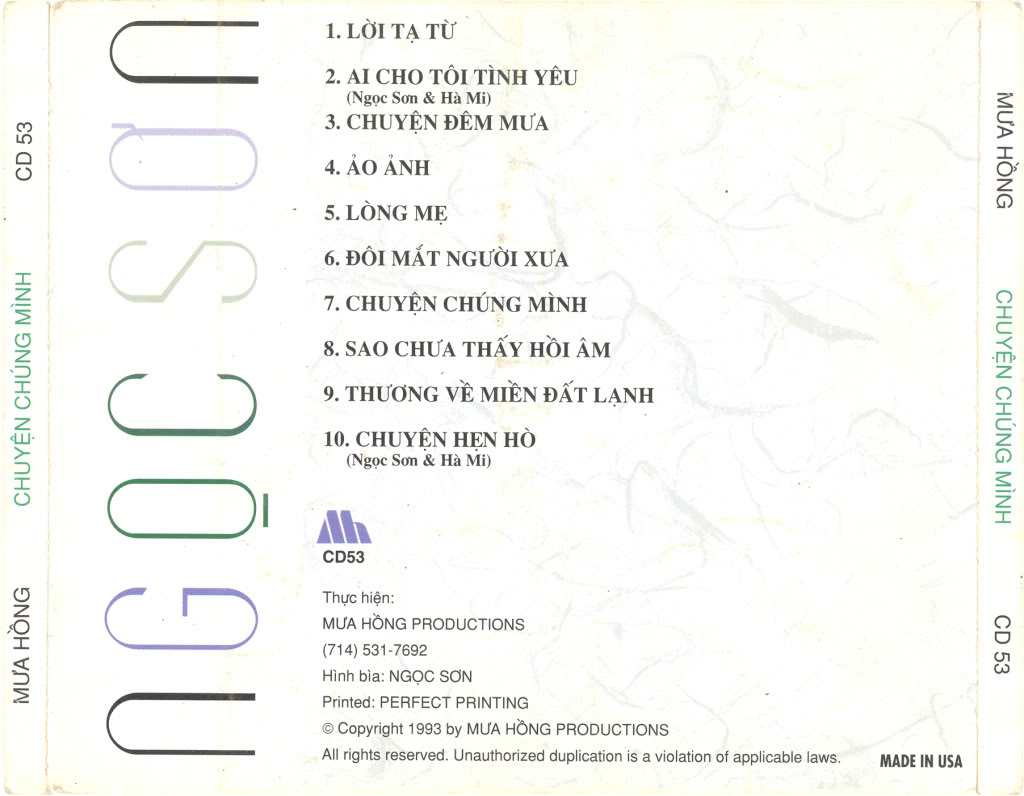The rectangular image appears to be the back cover of a CD case, resting on off-white paper embellished with grey flecks and yellow designs, giving it a vintage aesthetic. The standout title, "NGOCSON," is prominently displayed in large fonts of black, purple, and green, running vertically from bottom to top on the left border, and bottom to top on the right border. Below this, on the main body of the cover, is a list of ten songs, numbered 1 through 10, written in black font. Further down, centered, is a purple CD logo alongside the identifier "CD 53."

On both the left and right spines of the CD cover, the names "Mua Hong" and "Shuyuan Zhongmin" along with "CD 53" are printed similarly to the main title. The spine's orientation is vertical from bottom to top on the left and top to bottom on the right. Below the song list, additional fine print includes details such as "Mao Hong Productions," a contact phone number, and a copyright notice, specifying the production company, and "Made in USA," with a note of the printing by Perfect Printing and a 1993 copyright date.